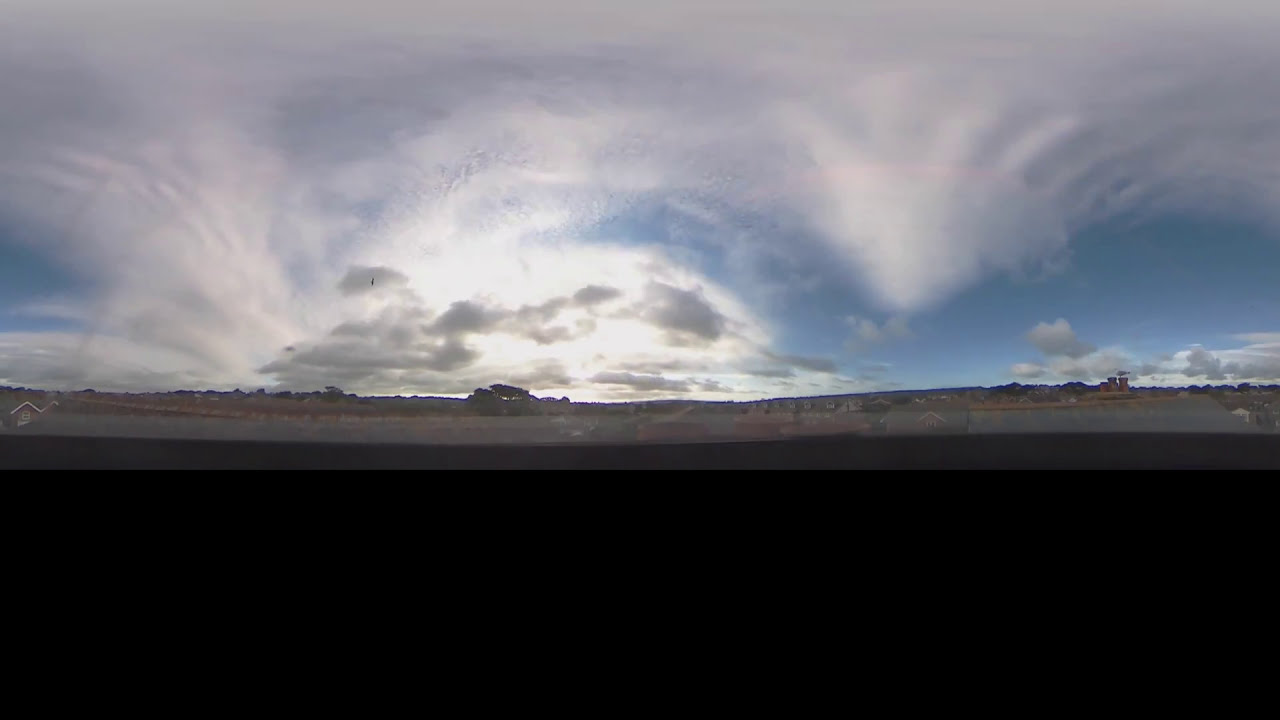The image captures a striking scenic view featuring an expansive sky that dominates the top half of the frame. The sky is a vibrant blue, adorned with unique, swirling cloud formations that transition into larger, wispy white clouds. Toward the horizon, the clouds become darker and heavier, casting a dramatic contrast. The sun, although hidden behind the clouds, illuminates the scene with a diffused light. 

Below this active sky, the middle section of the image reveals a hazy, distant horizon where several buildings, possibly houses, an apartment complex, or a condo, dot the landscape. There are smokestacks emitting small plumes of smoke to the right, and trees are visible on the far left, adding to the rural feel. The ground beneath this horizon appears barren, possibly dirt or sand, and features a road that stretches from the left side to the right, cutting through the terrain.

The bottom third of the image is a stark black rectangle, which is not a visible part of the landscape but rather a solid, opaque area that frames the picture.